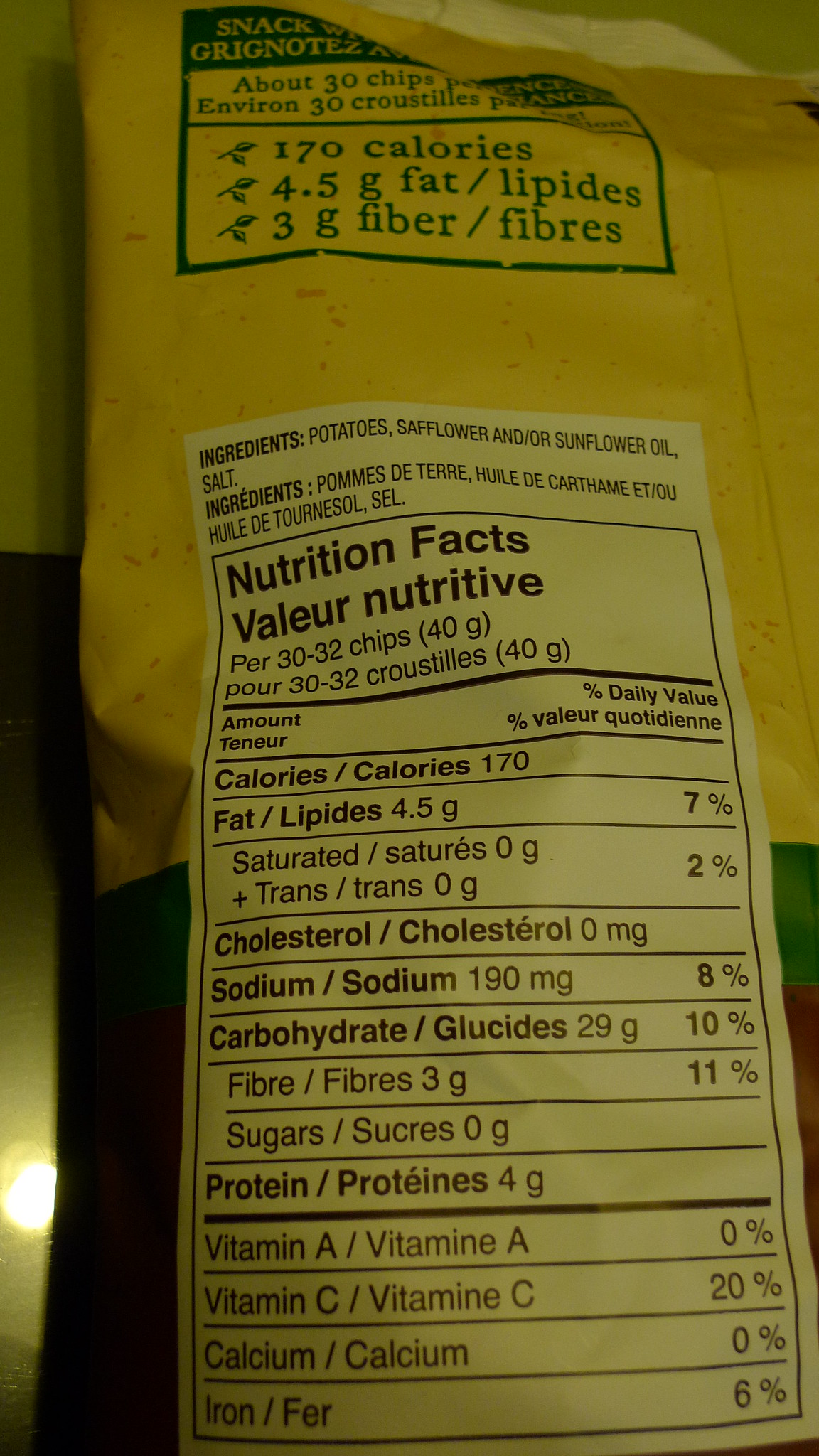The photograph depicts a nutrition label on a bag, which appears to be predominantly yellow with possible accents of brown or black, although the image is quite dark, making it challenging to discern the exact colors. The label indicates that the product inside the bag is chips, specifying nutritional information based on a serving size of 30 to 32 chips. The ingredients listed are potatoes, safflower or sunflower oil, and salt, confirming that the contents are indeed a type of potato chip. The nutrition facts are clearly displayed on the label, providing detailed information for consumers.